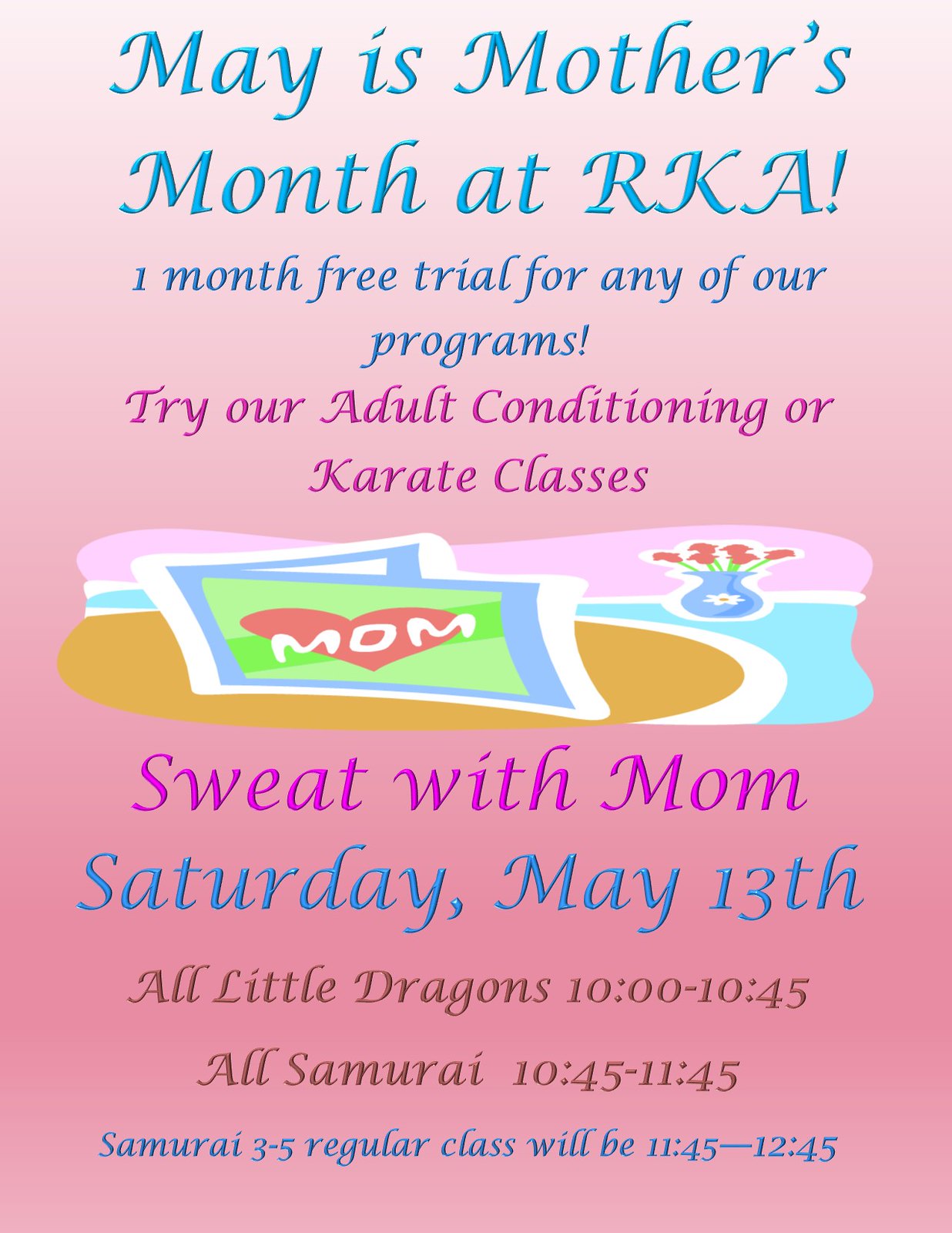The poster has a gradient pink background that transitions from light pink at the top to dark pink at the bottom. At the top in blue font, it reads, "May is Mother's Month at RKA." Below that, in a darker blue font, the text offers “One month free trial for any of our programs.” Further down, in magenta, it encourages attendees to “Try our adult conditioning or karate classes.”

The poster features an image depicting a cozy home scene: a blue floor with an orangey rug, a vase with red flowers, and a white pillow with a blue border, a green stripe, and a red heart that says "Mom." Beneath this image, in magenta, is the phrase "Sweat With Mom," followed by detailed scheduling information in blue font: "Saturday, May 13th," with activities for different age groups. "All Little Dragons: 10:00 to 10:45," in dark brown font, and "All Samurai: 10:45 to 11:45," followed by "Samurai 3-5 regular class: 11:45 to 12:45."